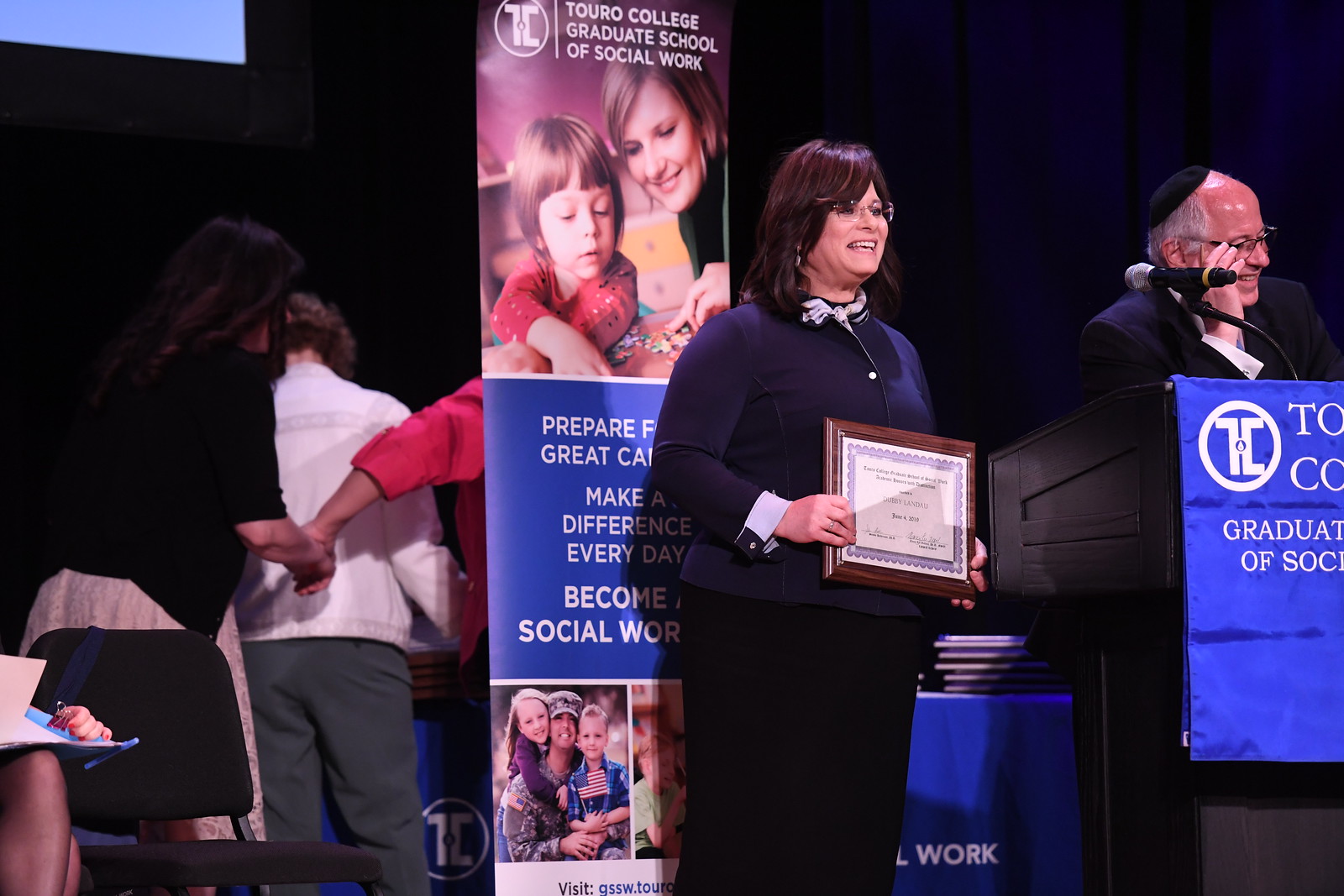In this indoor photograph, we are viewing a graduation ceremony held on a stage with a predominantly black background. The focal point of the image is a woman standing center stage, holding a dark wood-framed diploma. She has short brown hair, glasses, and is dressed in a long-sleeved blue shirt and a black skirt. Her expression is one of pride as she looks straight ahead at the audience. 

To her right stands a black wood podium adorned with a blue banner featuring partially visible white text, including the words "Graduate of Society." Behind this podium, an older man of Caucasian descent, possibly a rabbi, is laughing and smiling. He is wearing a black yarmulke and glasses, with his right hand raised near his face.

On the left side of the stage, a large rectangular banner with the text "Touro College Graduate School of Social Work" displays images of people working with children, along with the inspirational phrases, "Prepare Great, Make a Difference Every Day, Become Social Work." In the foreground on the left, three individuals, including two women who appear to be clasping hands, are walking away from the stage, presumably having just received their diplomas. 

The overall setting conveys the joy and achievement of the graduation ceremony.